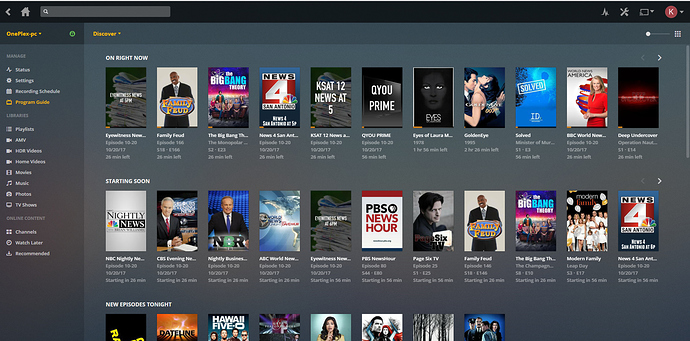The image showcases a streaming application interface, likely named OnePlex PC, displaying a variety of available movies and TV shows. The interface menu on the left side features several categories: Manage, Status, Settings, Recording Schedule, and Program Guide, with the Program Guide highlighted in orange, indicating it's currently selected. The options within the menu include Playlist, AMV, HDR, Home, Videos, Movies, Music, Photos, TV Shows, Channels, Watch Later, and Recommended. 

At the top, the interface includes a home button, a search field, and tool icons, along with a screen option and a KSI red circle situated in the upper-right corner. The main display area is divided into sections: "On Right Now," "Starting Soon," and "New Episodes Tonight." 

In the "On Right Now" section, various shows are listed against a gray background, including News, Family Feud, The Big Bang Theory, Channel 4 News, KSAT 12, QBee Prime, Eyes, GoldenEye, Solved, Something of America, BBC World America, and Deep Undercover. 

"Starting Soon" features a second row of options, some of which are repeats from the "On Right Now" section. 

At the bottom, the "New Episodes Tonight" section displays eight different shows, though the text is difficult to read. 

Overall, the application interface is filled with numerous entertainment options, providing a comprehensive guide to current and upcoming shows.